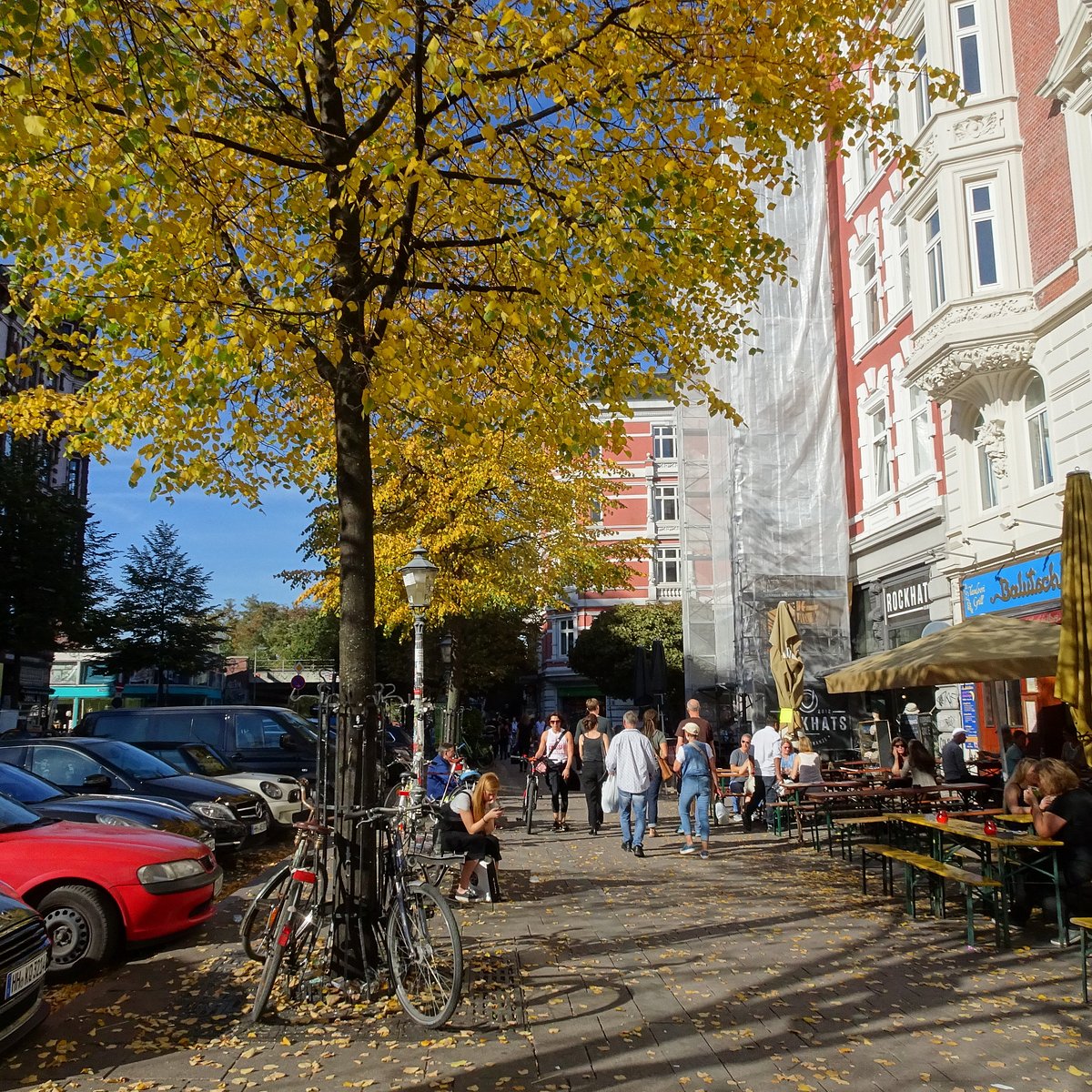The image depicts a lively urban courtyard on what seems to be a pleasant spring or fall day, characterized by trees with green and yellow leaves, some of which have fallen to the ground. On the left side of the courtyard, there is a parking lot with multiple cars facing the area. In front of one of the trees, two bikes are parked on each side, suggesting a designated bike rack area. A small lamppost stands next to a bench between the two trees, where people are casually seated. 

To the right side of the courtyard, several benches with umbrellas provide shaded seating for people who are engaged in conversation and enjoying drinks, indicating nearby retail shops or cafes. A person can be seen pushing a bike along a path, contributing to the scene's dynamic atmosphere. Dominating the background are tall buildings, one of which is white and brown, while another resembles a college building. These structures suggest a mixed-use space, creating a harmonious blend of leisure, retail, and residential areas.